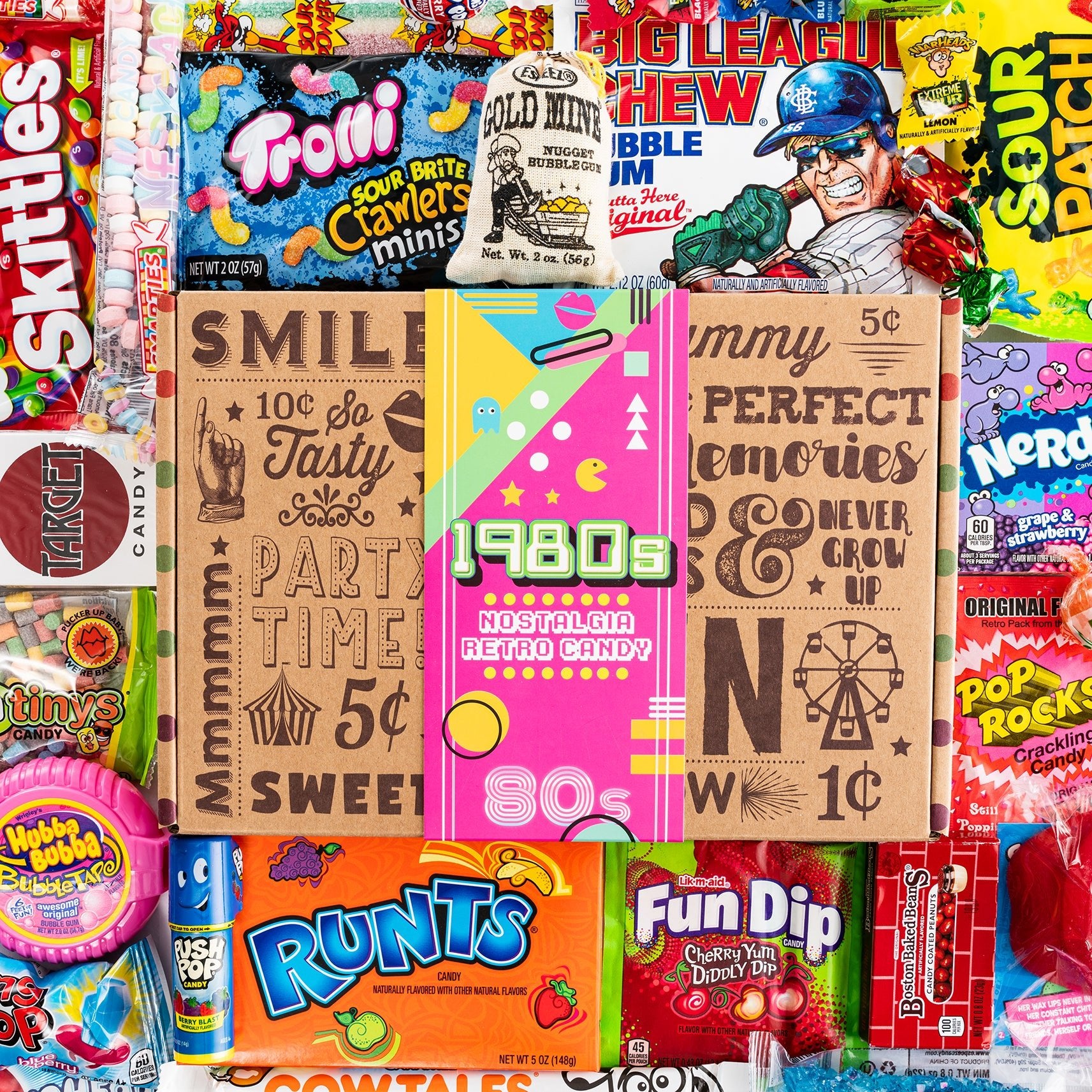The image is a vibrant tribute to 1980s nostalgia, centered around a colorful banner that reads "1980s Nostalgia Retro Candy" in a playful arcade-style font. The banner features iconic 80s imagery, including a yellow Pac-Man and a blue ghost, and is wrapped with a tan ticket adorned with partial words like "Smile," "Perfect," "Tasty," "Party Time," "Five Cents," "Ten," and "One Cent," evoking a retro feeling. Surrounding the banner is a cornucopia of classic candies. At the bottom left, we spot a pink roll of Hubba Bubba gum, a blue-packaged Ring Pop, and a blue Push Pop. Adjacent to these are an orange box of Runts, a packet of Fun Dip, and various other candies like Pop Rocks, Nerds, Trolley, and Skittles. The upper section showcases Sour Patch Kids, Big League Chew, and Sour Brite Crawlers. A cardboard box in the background, featuring words like "Party Time" and "Tasty," adds to the nostalgic ambiance. The left side also features a candy necklace and a white-packaged candy with a red circle, further enriching this vibrant collage of 80s candy nostalgia.